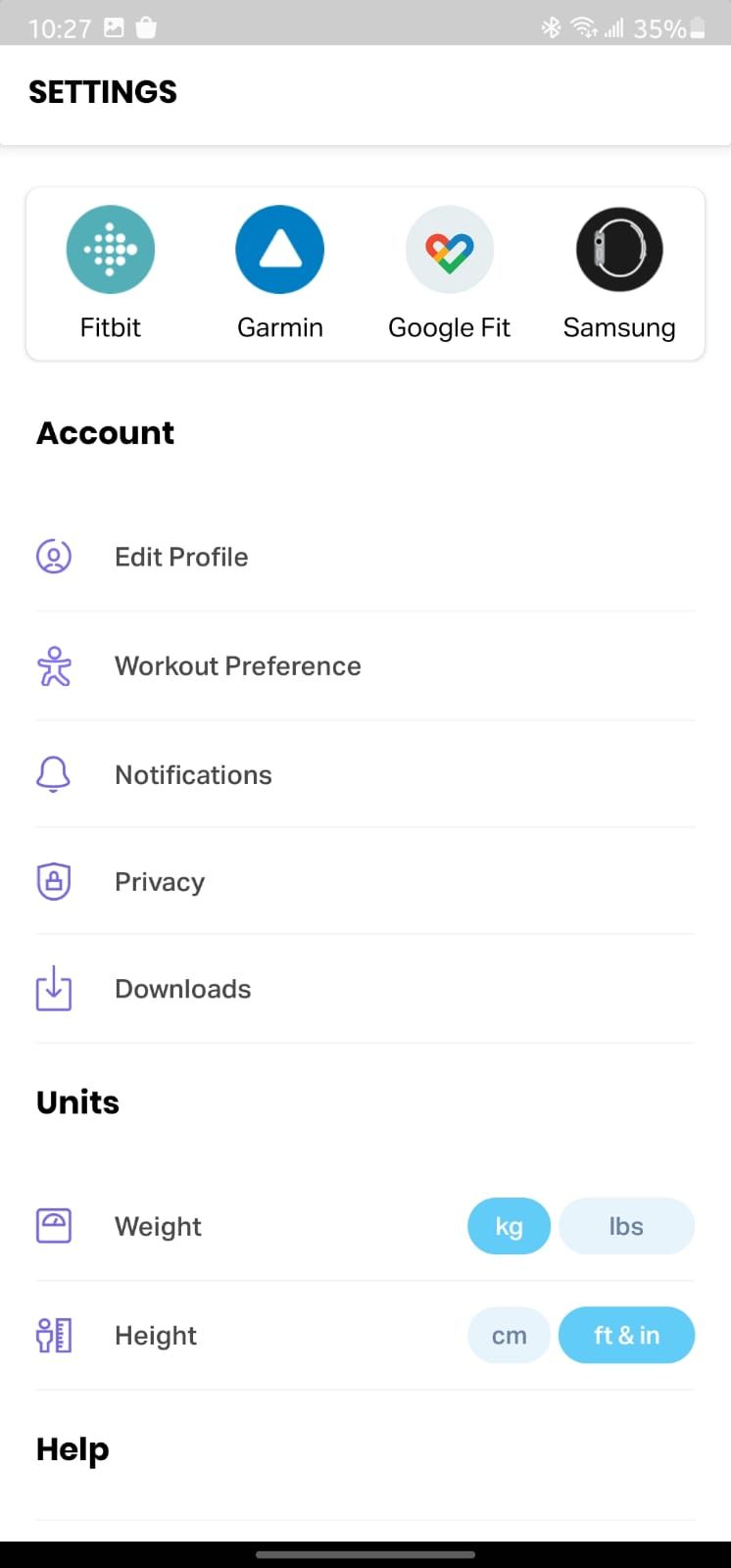This screenshot captures a mobile device's settings page at 10:27 AM, as indicated by the clock displayed on the top left corner. The status bar at the top of the screen showcases an active Bluetooth connection, full Wi-Fi signal strength, active download and upload icons, full network signal strength, and a battery level at 35%. 

The settings page includes the following options: "Settings," "Fitbit," "Garmin," "Google Fit," "Samsung," "Account," "Edit Profile," "Workout Preference," "Notifications," "Privacy," "Downloads," "Units," and "Weights." Notably, the weight metric is set to kilograms rather than pounds, and the height metric is set to feet and inches instead of centimeters. Additionally, the interface features "Help," and the navigation buttons are displayed on a slim black bar at the bottom of the screen.